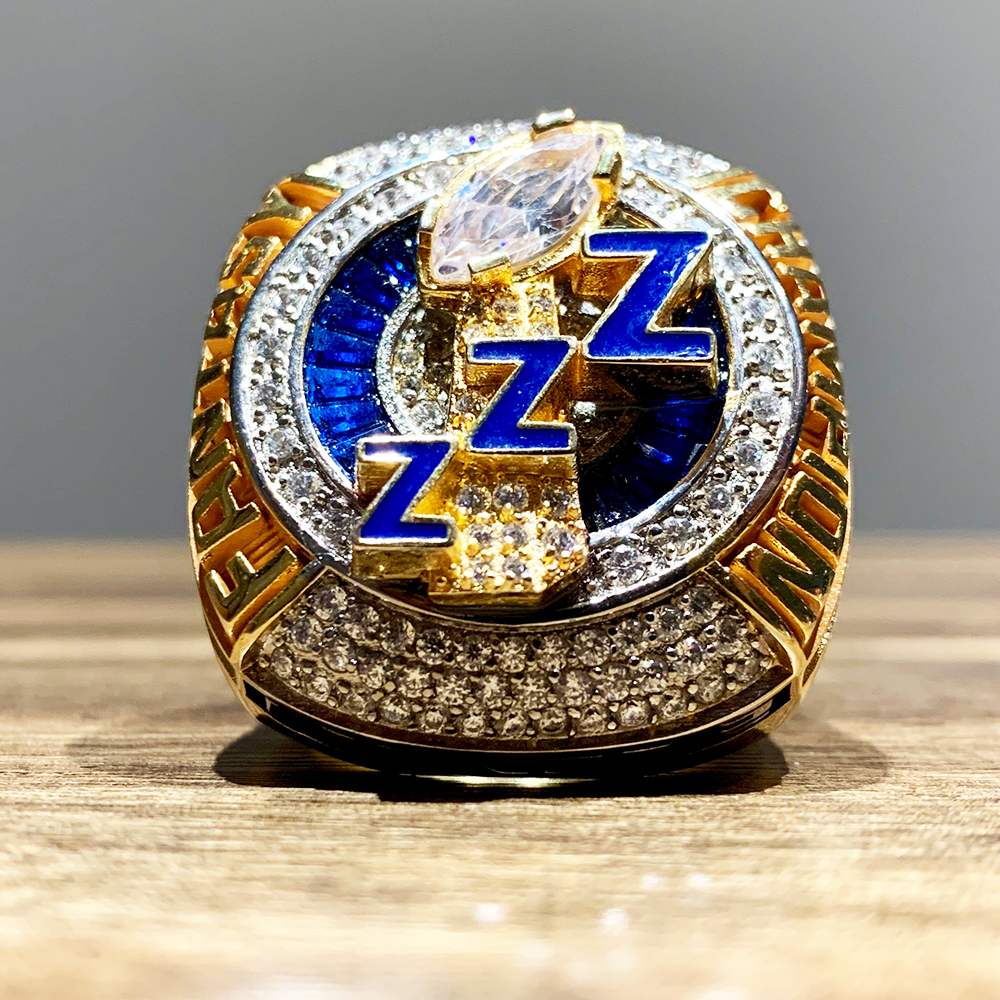An exquisitely detailed photograph captures a champion's ward-style ring resting on a light green wooden surface, set against a gray wall backdrop. The ring is an opulent creation of gold and diamonds, featuring intricate engravings on either side. The left side proudly displays the word "Fantasy" in gold letters, while the right side proclaims "Champion." Rows of sparkling diamonds adorn both the top and bottom borders of the ring. At the ring's center lies a dazzling array of pavé-style diamonds encircling a clear-cut diamond shaped like a football, perched on an elegant diamond and gold pedestal. This stunning centerpiece is crowned with three vivid cobalt blue Z's, set atop a row of rectangular cut sapphires, adding a majestic touch to this remarkable piece of jewelry.